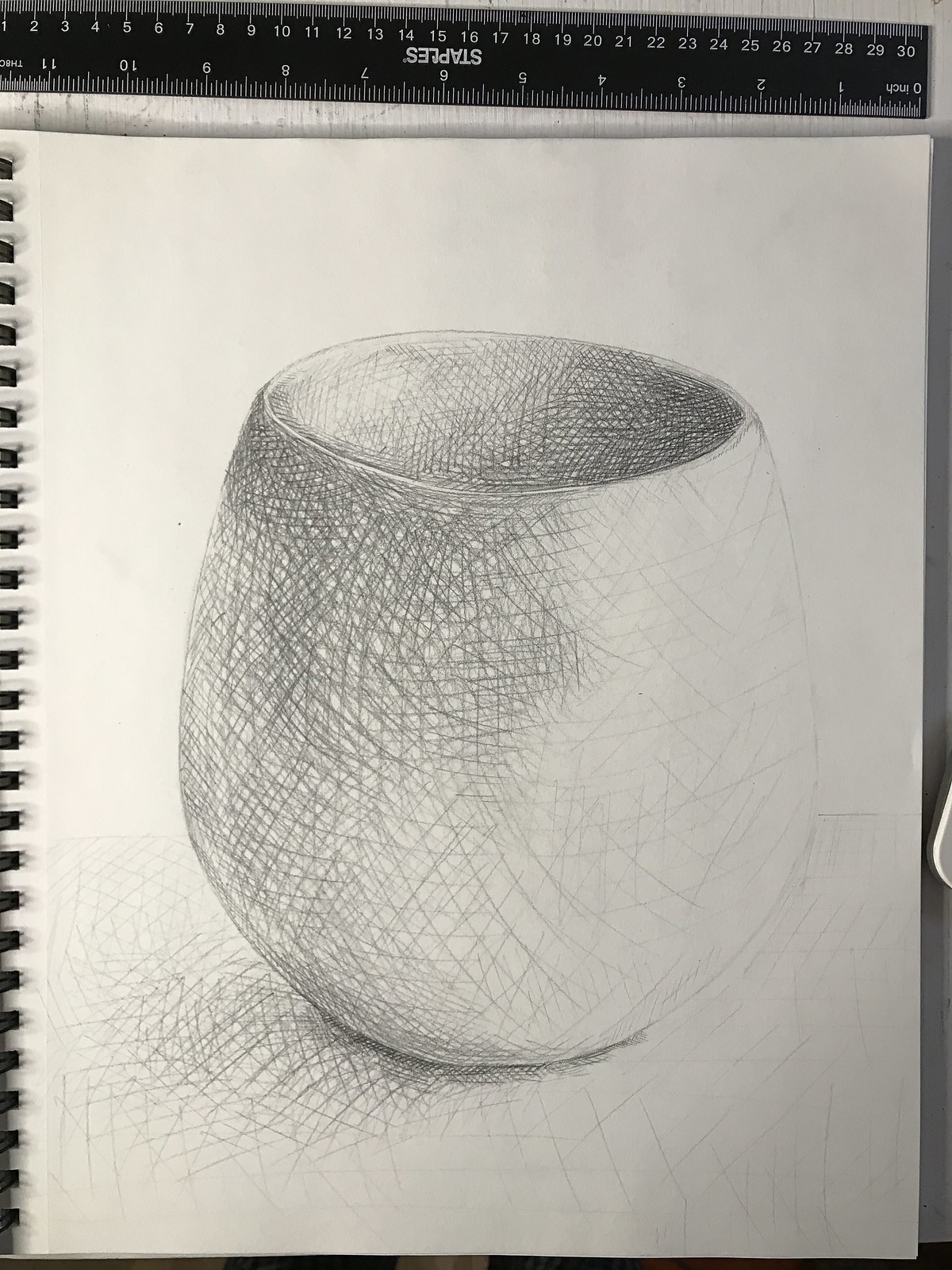This is a photograph of an open sketchpad. On the right page of the sketchpad, there is a detailed pencil drawing of a vase. The vase has a rounded, almost globe-like shape, with meticulous crosshatching and hash marks primarily used for shading. The left side of the vase is heavily shadowed with darker cross marks, indicating the light source is coming from the right side, which is much lighter in shading. The vase also features some round lines at the opening and bottom, enhancing its three-dimensional appearance. 

The sketchpad has a white background, and the black spiral binding is visible along the left edge of the page. Additionally, at the top of the image, there is a black ruler with white writing and numbers, branded with "Staples," positioned upside down. The shadow of the vase extends towards the bottom left onto the table where the sketchpad rests, also depicted with crosshatching. This pencil drawing on a notebook pad appears to be a detailed study piece, indicative of a beginner artist mastering shading techniques.